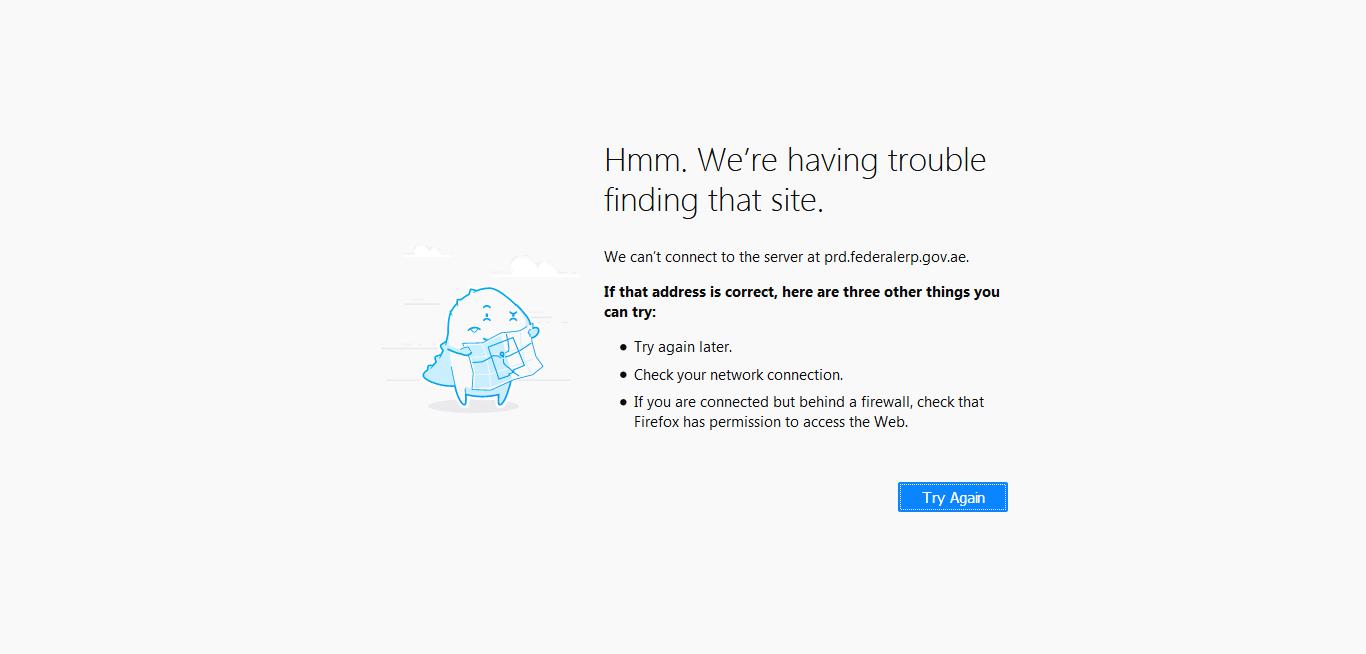This image captures an error page encountered when trying to access a website, characterized by its light gray background. In the center of the page, there is a blurb with left-aligned text that features an icon on its left side, positioned at the lower part of the blurb. The icon resembles a blue silhouette of a creature that appears to be a hybrid between a bear and a dinosaur, holding what looks like a map. The creature has two pointy legs and a small tail.

To the right of the icon, the blurb reads: "Hmm. We're having trouble finding that site." Below this sentence, in smaller font, it states: "We can't connect to the server at PRD.federal.erp.gov.a". Underneath this, the text continues: "If that address is correct, here are three other things you can try:" followed by three bullet points.